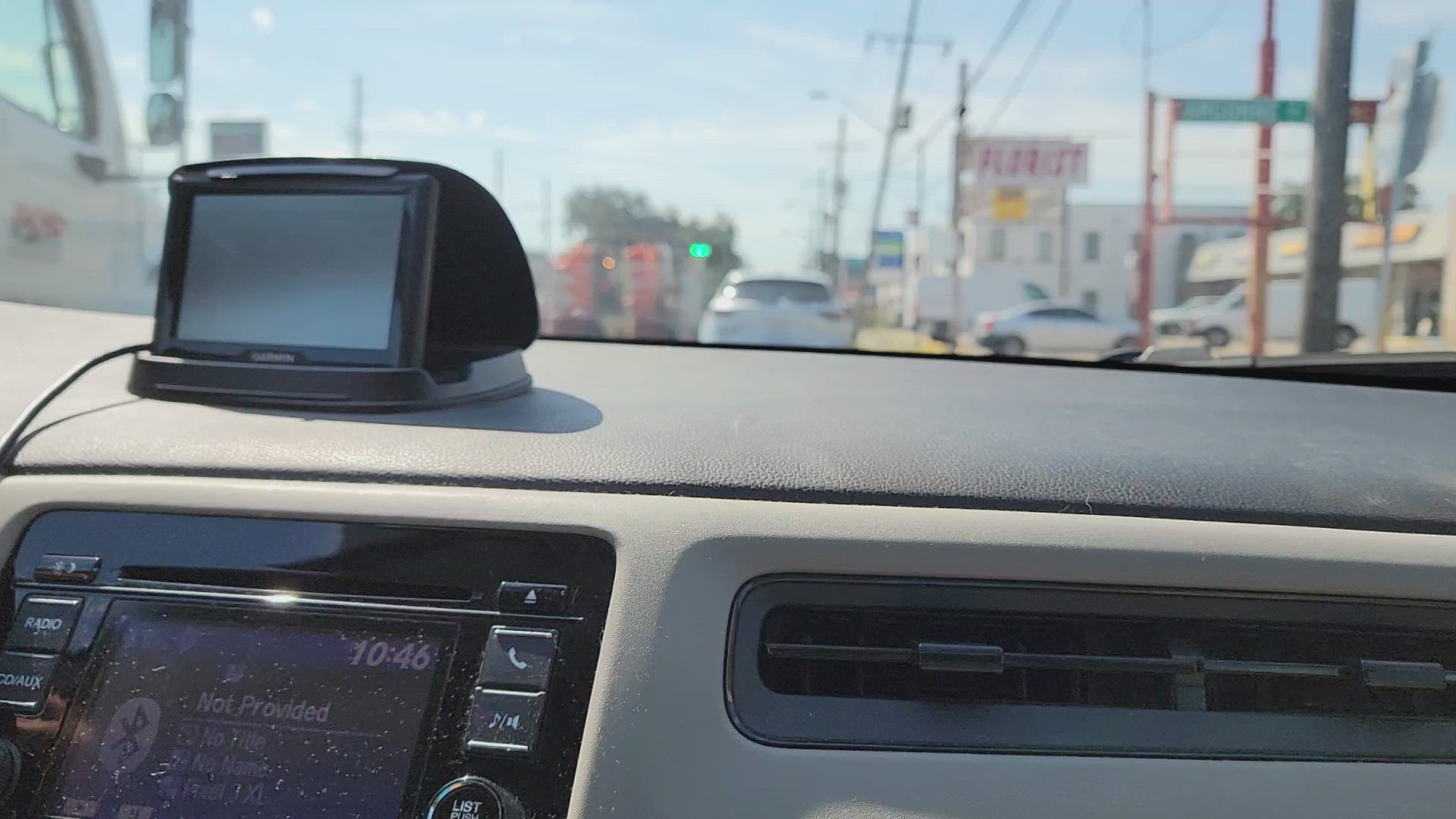This image captures the perspective from a car's driver seat, focusing on the dashboard and the view through the windshield. The dashboard features a mix of black and grey tones, with a striking black top and a grey console area accented by black trim. Prominently mounted on top is a Garmin GPS unit, presumably directing the journey. The car's digital display shows a Bluetooth connection screen with the time reading 10:46 AM, illuminated by bright sunlight. The screen is slightly dusty, indicating that it is not currently playing music via Bluetooth. 

There are a variety of buttons visible on the console, including those for radio, CD-AUX, calls, and music volume control. Just to the right of these buttons is a sleek, slim-line AC vent. 

Through the windshield, the road ahead is slightly blurred, giving a sense of motion. Several vehicles, including a couple of white cars, can be seen driving ahead, while a few cars are parked on the right side of the road. The image conveys a typical driving scenario on a sunny day.